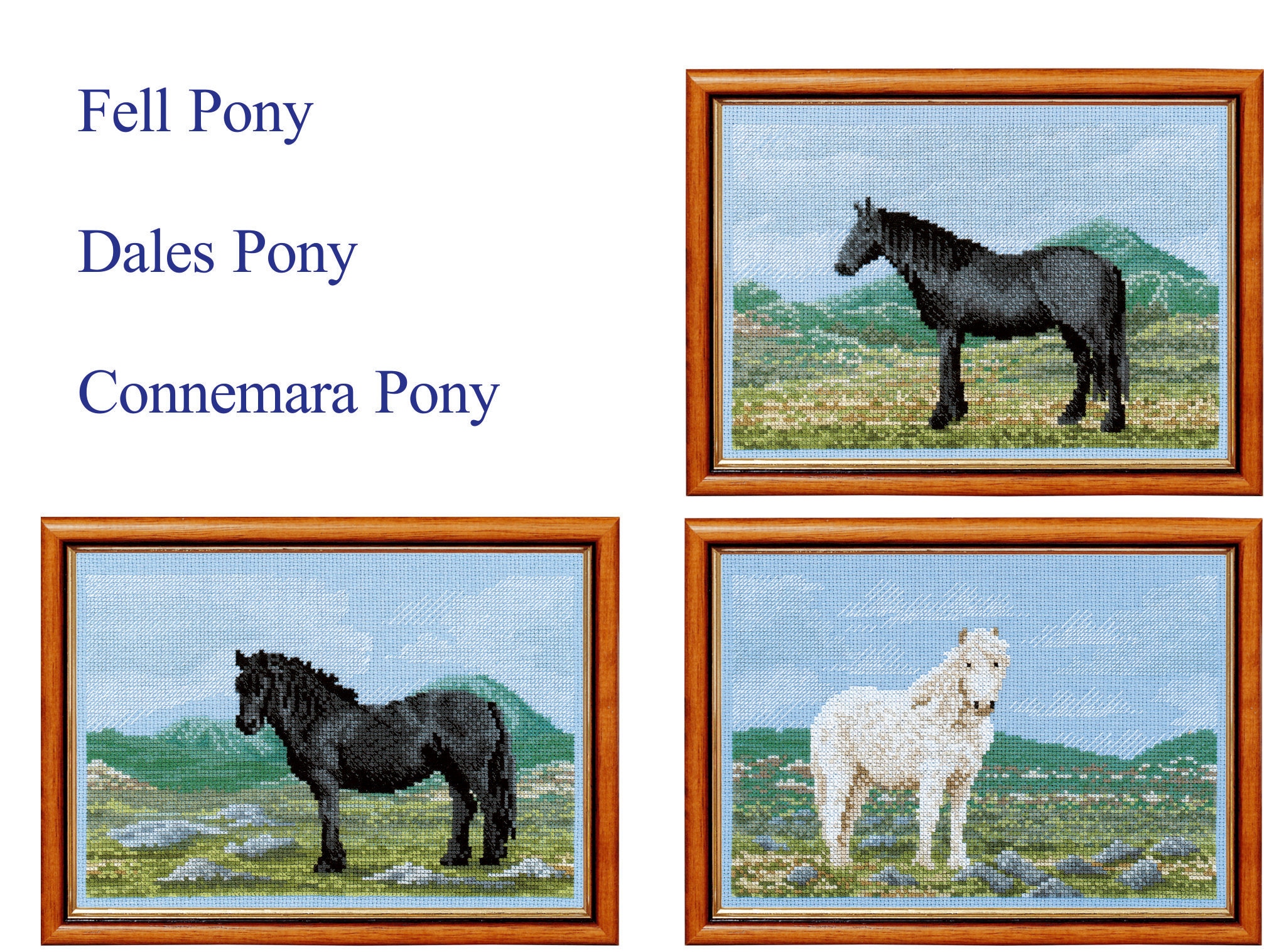The image features three framed needlepoint depictions, each highlighting a different pony breed: the Fell Pony, the Dales Pony, and the Connemara Pony. Each pony is individually framed with a brown frame, set against a white background with their breed names inscribed in blue letters. The top left frame hosts the Fell Pony, a black horse standing beside a small hill under a clear blue sky, with green mountains in the background. The bottom left frame displays the Dales Pony, another black horse of similar appearance, also positioned in front of a hilly/mountainous landscape. The right frame features the Connemara Pony, a striking white horse facing forward amidst a similar serene setting. All ponies appear in a heather field dotted with rocks, and the embroidery work is notably crude, giving the images a pixelated look due to the large stitches.